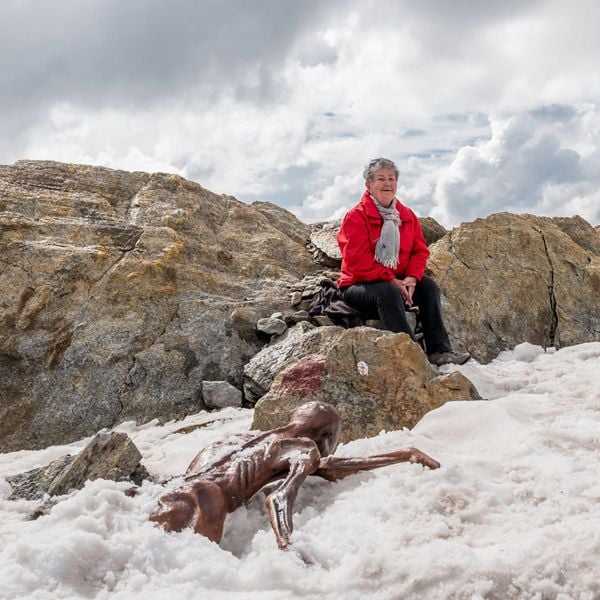In this mesmerizing daytime photograph set amidst a cold, snowy landscape with expansive white clouds and towering, mountainous rocks, an older white woman, sporting short gray hair, sits serenely on a large rock. Dressed warmly in black pants, a red coat, and a white scarf, she smiles gently at the camera. The snow-covered ground at her feet adds to the chilly ambiance. In stark juxtaposition to her calm demeanor, a mummified body with brown, desiccated skin lies face down in the snow nearby, its arms outstretched as if in mid-climb. The haunting figure, which resembles a skeleton with a dark red tinge, seems to be crawling out of the snow towards her, creating an eerie yet captivating contrast against the tranquil, natural background.